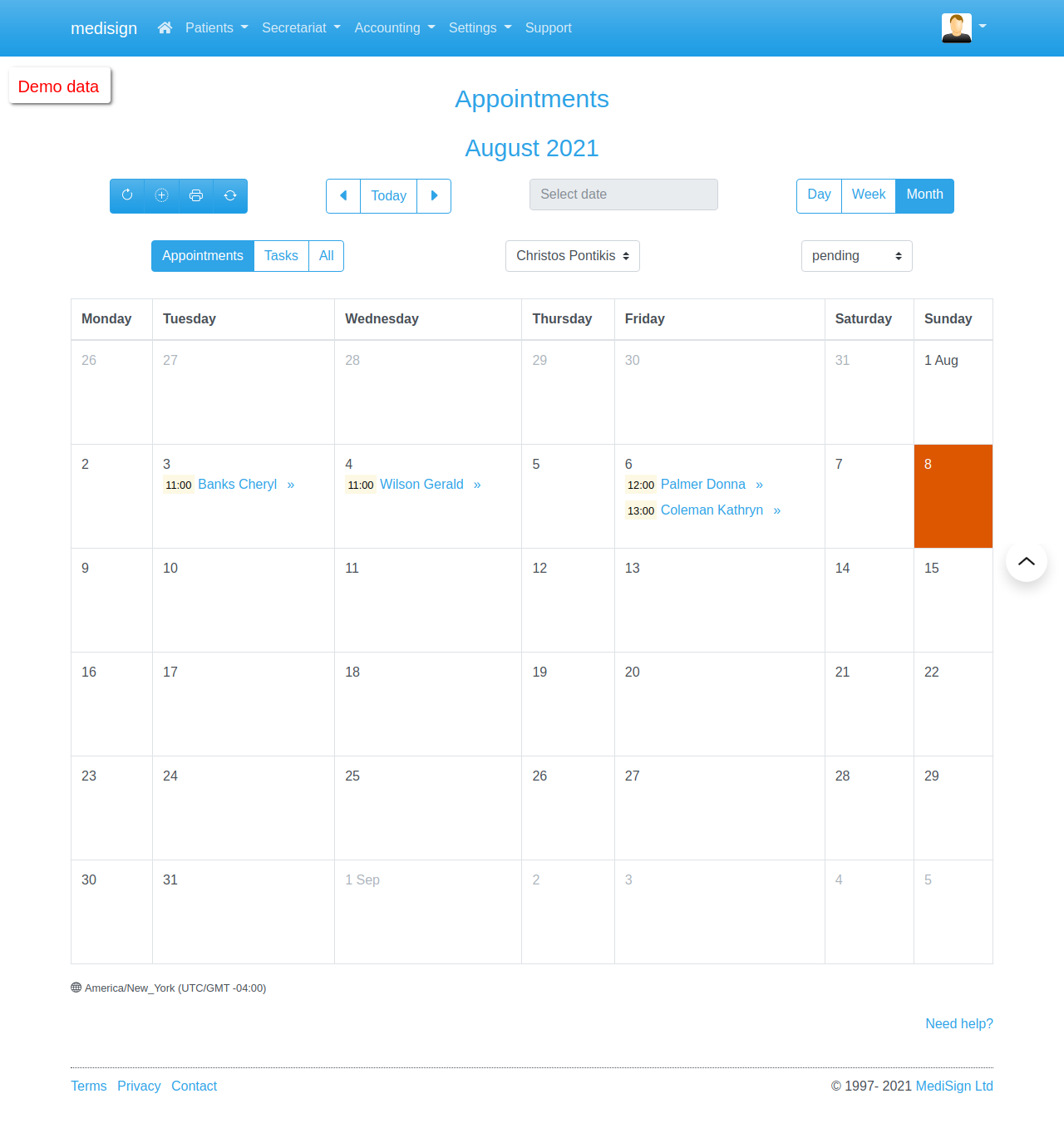The image showcases a detailed interface, predominantly in shades of blue and white. At the top, a large blue header prominently displays the word "Medicine." This header also features various white labels with downward arrows next to them, indicating dropdown menu options. Adjacent to these labels is an icon of a person accompanied by another downward arrow.

Below the header, there is a small white button with the text "Demo Data" written in red. Centrally located on the page is a label that reads "Appointments in August 2021." Beneath this, there is another blue section adorned with various small icons.

Subsequently, there's a box labelled "Today," which is flanked by left and right arrows for navigation. Another blue box contains the label "Select Date," and below it, there are three distinct smaller boxes marked "Day," "Week," and "Month."

Further down, the interface is segmented into categories for "Appointments," "Tasks," and "All," followed by specific entries such as "Chrysalis" and "Pancus," each with a "Pending" status. A calendar layout is displayed next, detailing appointments for the month. The entries include:
- On the 3rd at 11:00 AM: "Banks Cheryl"
- On the 4th at 11:00 AM: "Wilson Gerald"
- On the 6th at 12:00 PM: "Palmer Doris"
- On the 6th at 11:00 AM: "Catherine" (first name obscured)
- On the 8th: a significant orange box, indicating an important event for the day

Additionally, a small circle with an upward arrow appears near the orange box, seemingly for additional actions.

At the very bottom of the interface is a small blue circle with accompanying text, and on the right side, there is more textual information in blue print, ending with a blue box that contains the years "1997 to 2021."